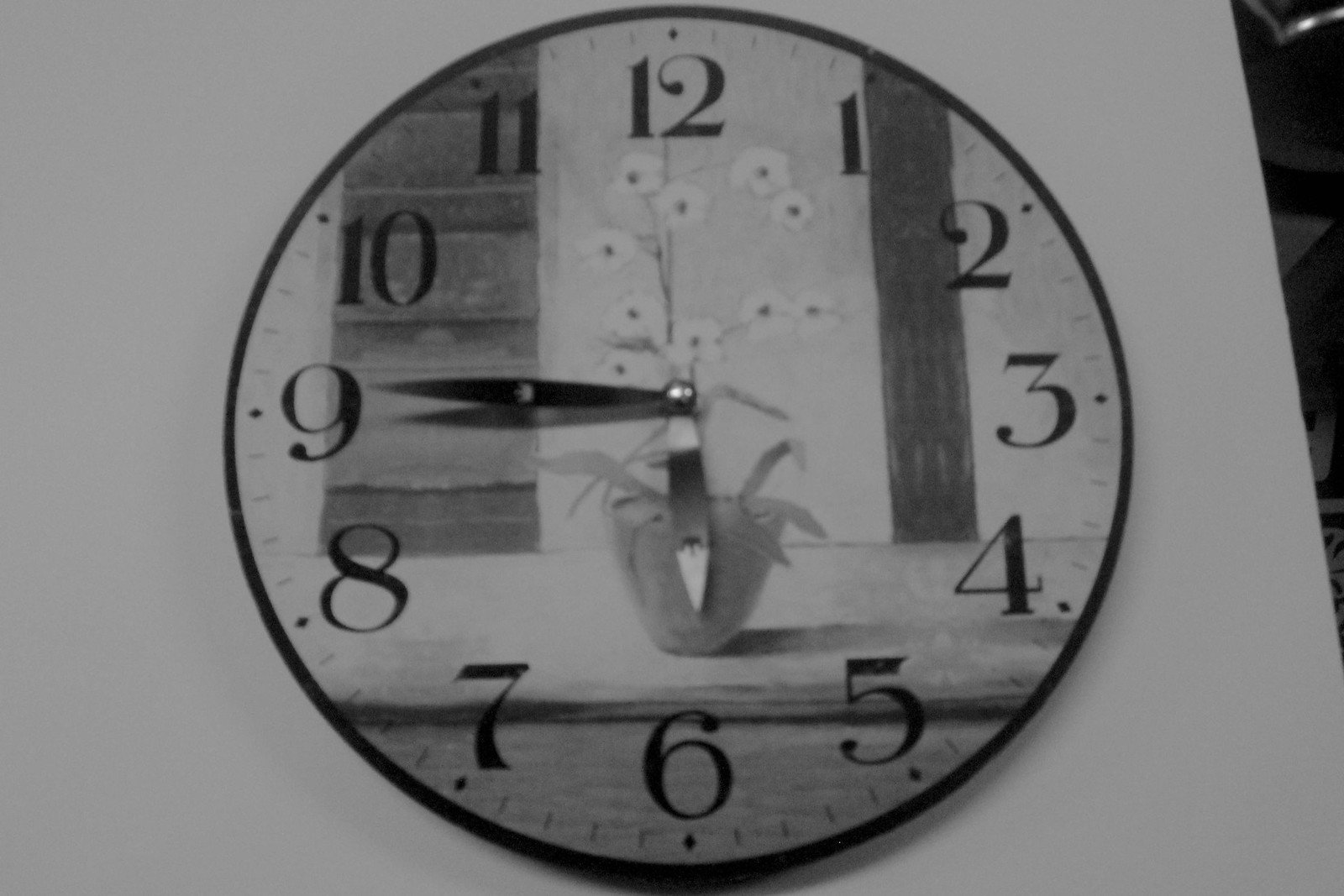This black and white photograph or drawing features a vintage, round clock with bold black numerals from 1 to 12. The clock's face is adorned with an intricate illustration of a potted plant, complete with blooming white flowers that have distinctive black centers. The plant, in its decorative planter, is positioned centrally on the clock, with larger lines extending through the numerals from 11 to 4. The clock itself is outlined in black and rests on what appears to be a white table, amidst a simplistic backdrop that resembles a bookcase. The clock's sharp, metallic hands, secured by a small circular bolt, indicate the time as 14 minutes to 6. This detailed scene is entirely rendered in shades of gray, black, and white, emphasizing the contrast and timeless elegance of the piece.